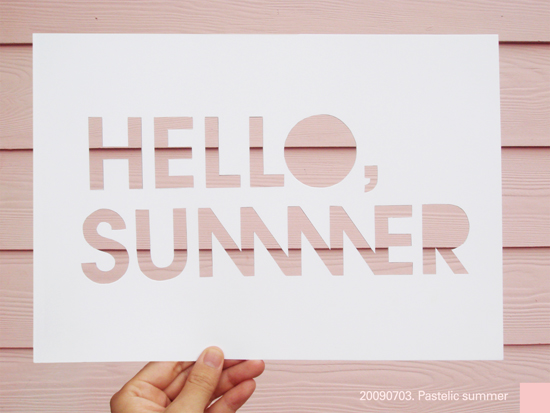The image depicts a left hand holding a white piece of paper against a background that resembles muted, wood-panelled pink house siding. The paper features cut-out letters revealing the pink background through them, forming the text "Hello, Summer" with a comma after "Hello," The top row of letters spells "Hello," while the bottom row spells "Summer." Near the bottom right of the paper, there's a watermark text that reads "20090703.pastelicsummer" alongside a pink square. This sign appears to be suitable decor for summer settings, such as a home, cottage, or beach house.